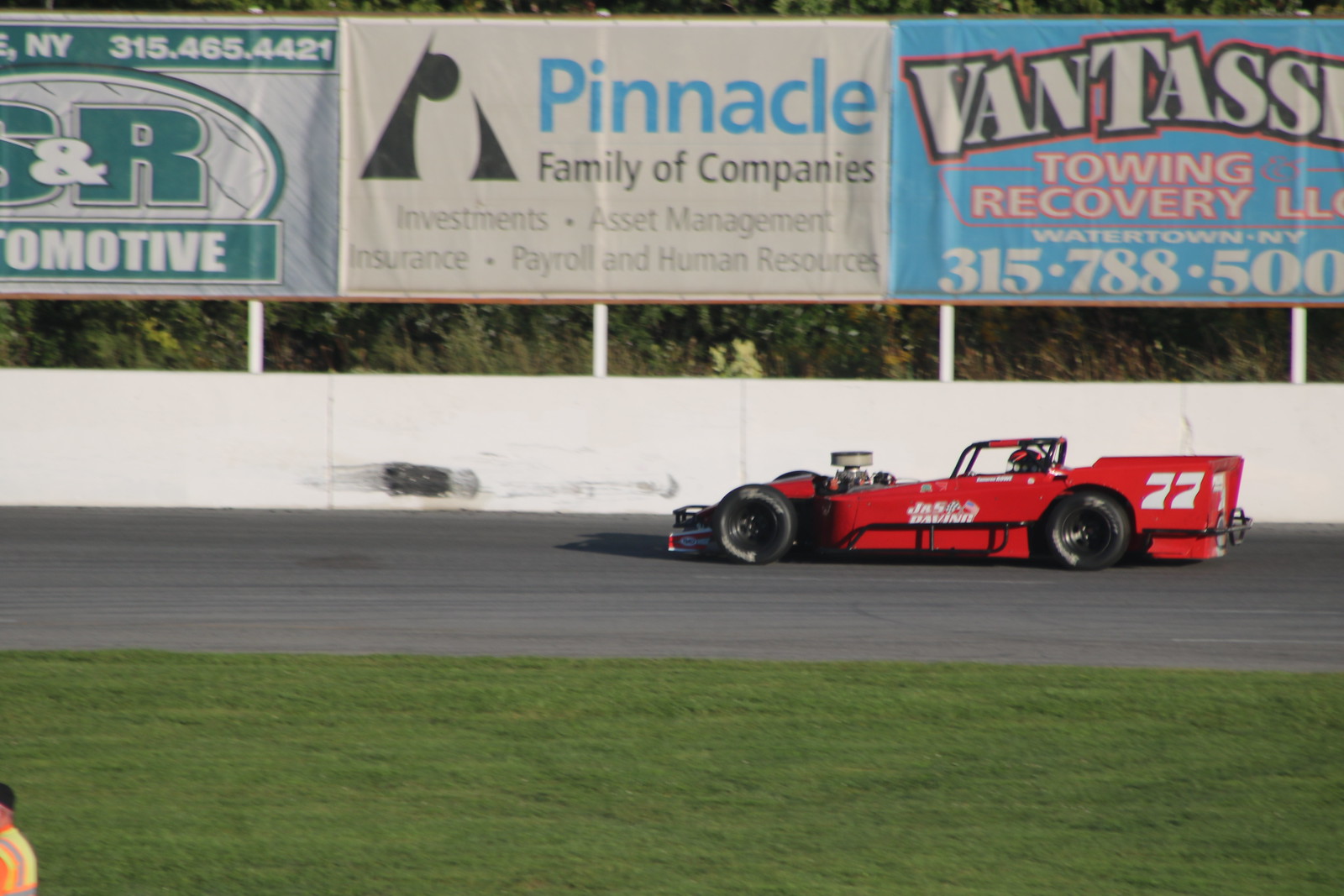This detailed image showcases a red Formula 1 race car, adorned with the number 77, racing on a gray asphalt track. The car, with its open cockpit and engine, is positioned on the right side of the image, driving towards the left. The track is bordered by a lush green grass inland field in the foreground and a white barrier wall, which shows black scuff marks, possibly from a previous collision, behind the car.

Above the barrier wall, there are three advertisement banners supported by white poles. The banner on the far left is green and white, promoting "SNR Automotive." The middle banner advertises "Pinnacle Family of Companies" and lists services including Investments, Asset Management, Insurance, Payroll, and Human Resources. The rightmost banner is for "Van Tass Towing Recovery LLC" located in Watertown, New York, with a partially visible phone number (315-788-500).

In the bottom left corner of the image, a person wearing a safety vest and a black cap can be seen from behind. The scene is further enriched by the presence of green trees and bushes in the background, adding depth to the raceway setting.